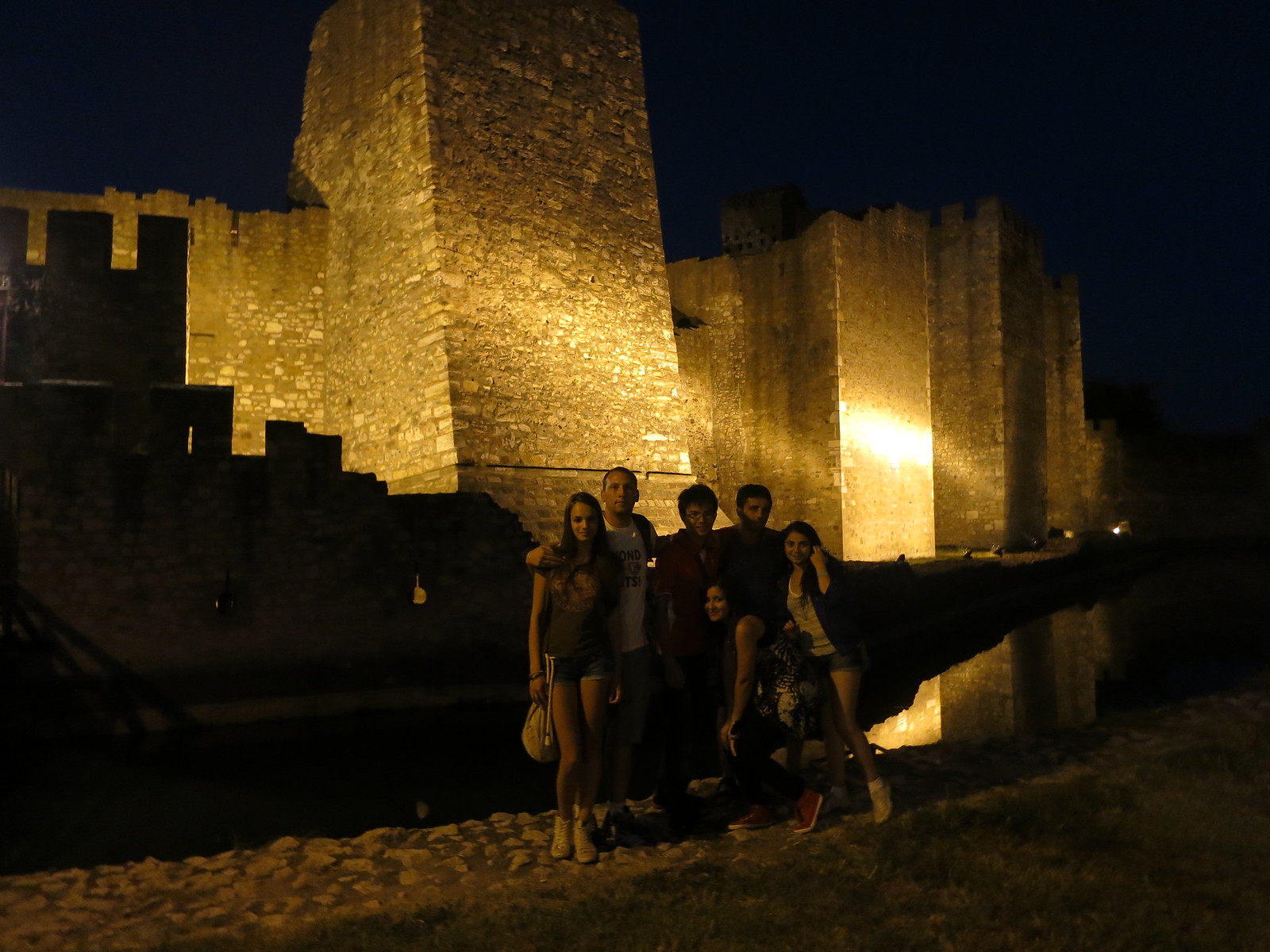In this captivating nighttime photographic image, a group of six people, including three women and three men, are standing outside in front of a grand historical structure that resembles an ancient monument or castle. The impressive edifice, characterized by its towering gray stone pillars and castle-like facade, reaches high into the dark sky. It is partially illuminated by golden light streaming through some of the pillars, casting a soft glow onto the group.

From left to right, the first person is a woman who appears to be Hispanic, dressed in shorts and white sneakers, carrying a bag and a shirt. To her right is a tall man who looks to be white, identifiable by his white shirt and his comforting hand resting on her shoulder. The next individual is a man whose features are cast in shadow, making it challenging to distinguish his ethnicity, but he appears to be either Black or Hispanic. Kneeling slightly in front of this man is a woman wearing red sneakers and pants. Behind her stands another woman, smiling with shoulder-length hair, dressed in shorts, white sneakers, and a jacket. Flanking the group on the far right is another man, similarly obscured by shadows.

The setting is further enhanced by a reflective puddle or canal to the group's right, capturing the ambient light and adding depth to the scene. In the background, a tall stone pillar rises prominently, signifying the central element of the monument. The group appears to be standing on a stone paved area, just a short distance from what seems to be a moat or drop-off, possibly hinting at an ancient fortification with a drawbridge nearby. Overall, the image conveys a sense of exploration, camaraderie, and historical intrigue against the magnificent nighttime backdrop.